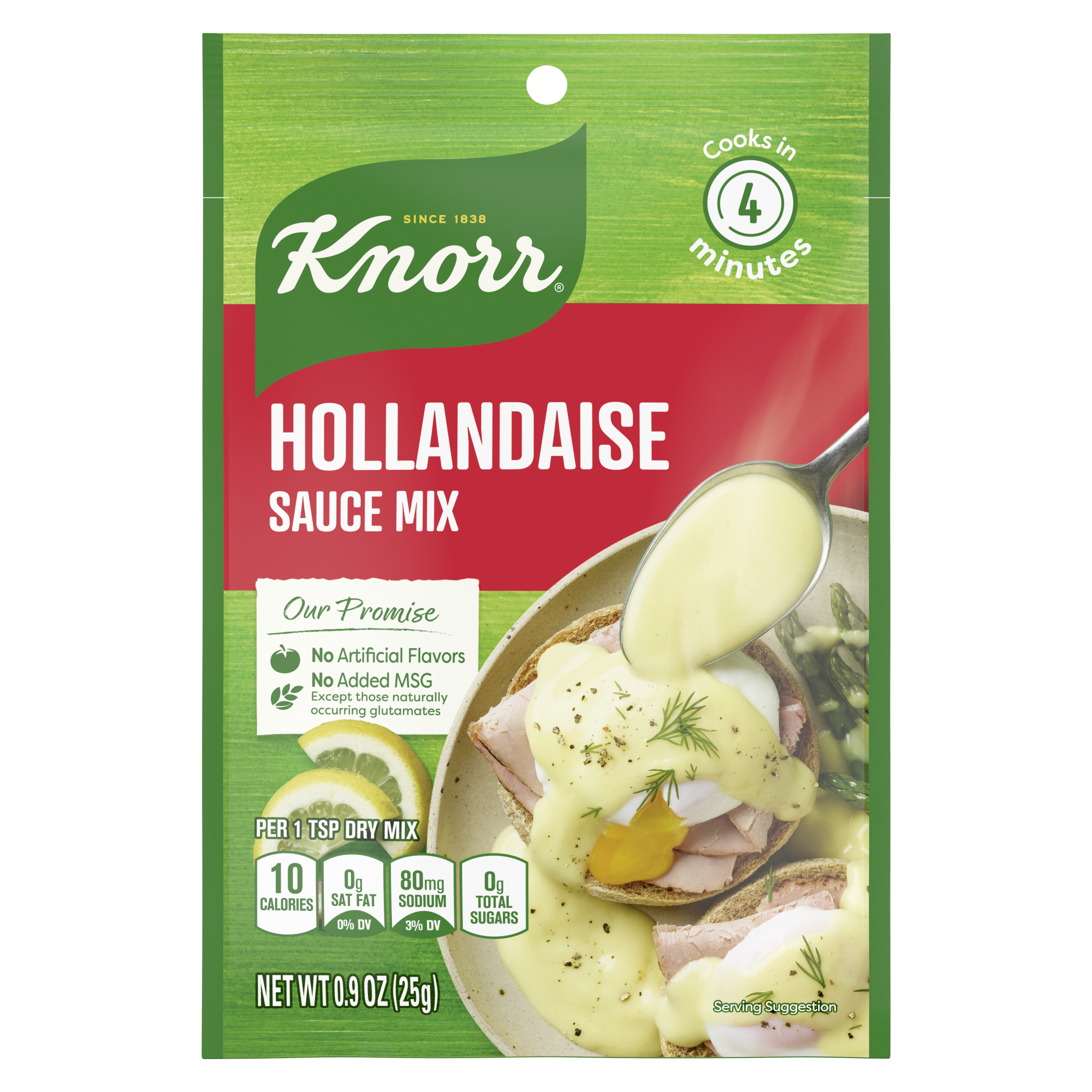The image shows the packaging for Knorr Hollandaise Sauce Mix, a product from a brand established in 1838. Promising to cook in just four minutes, this mix is marketed with the assurance of "no artificial flavors" and "no added MSG, except those naturally occurring glutamates." The package details nutritional information such as 10 calories, 0 grams of saturated fat, 80 milligrams of sodium, and 0 grams of total sugars per teaspoon of dry mix. The net weight is 0.9 ounces (25 grams). The vibrant packaging features a color scheme that includes light green, green, white, red, yellow, pink, and tan accents. 

The image also showcases a serving suggestion: an open-faced English muffin topped with ham, an egg, and a pour of creamy yellow Hollandaise sauce, accompanied by green beans on the right. These items are arranged on a plate with a spoon positioned above the English muffin. To the left, there are wedge slices of lemon, adding a fresh touch to the presentation. The design includes a small punch hole at the top, indicating it is intended for hanging on store shelves, reinforcing that this is a retail package design for the sauce mix.